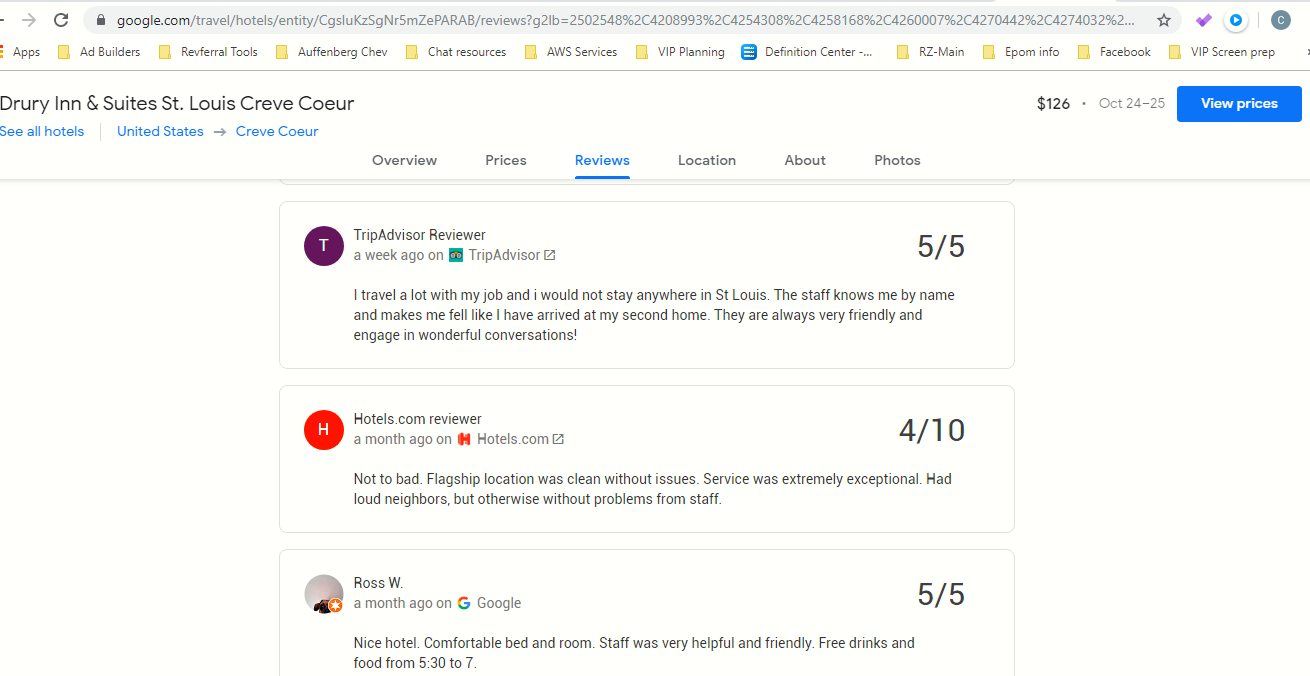This is a detailed screenshot of a Google Travel search results page for hotels. At the top of the page, there's a search bar indicating the URL: google.com/travel/hotels/entity followed by a series of letters and numbers. Below the search bar, there's a list of folders on the left side. These folders are labeled as apps, ad builder, referral tools, Kloffenberg chev, chat resources, AWS services, VIP planning, definition center, RZ main, EPUM info, Facebook, and VIP screen prep. A black line separates these from the main content area.

On the left-hand side, a heading reads "Jewelry Inn and Suites, St. Louis, Creve Coeur." To the right of this heading, the price of $126 is displayed for a stay from October 24th to 25th, alongside a blue button with white text that says "View Prices."

Directly beneath the hotel name, links are provided for navigating to additional hotel listings, labeled "See all hotels, United States," with Creve Coeur indicated by an arrow icon. The main content area presents several navigation options: Overview, Prices, Reviews, Location, About, and Photos, with the "Reviews" section currently selected, shown underlined and in blue.

The review section lists the first three reviews as follows: a TripAdvisor review with a rating of 5 out of 5, a Hotels.com review with a rating of 4 out of 10, and a review from "Ross W." with a rating of 5 out of 5.